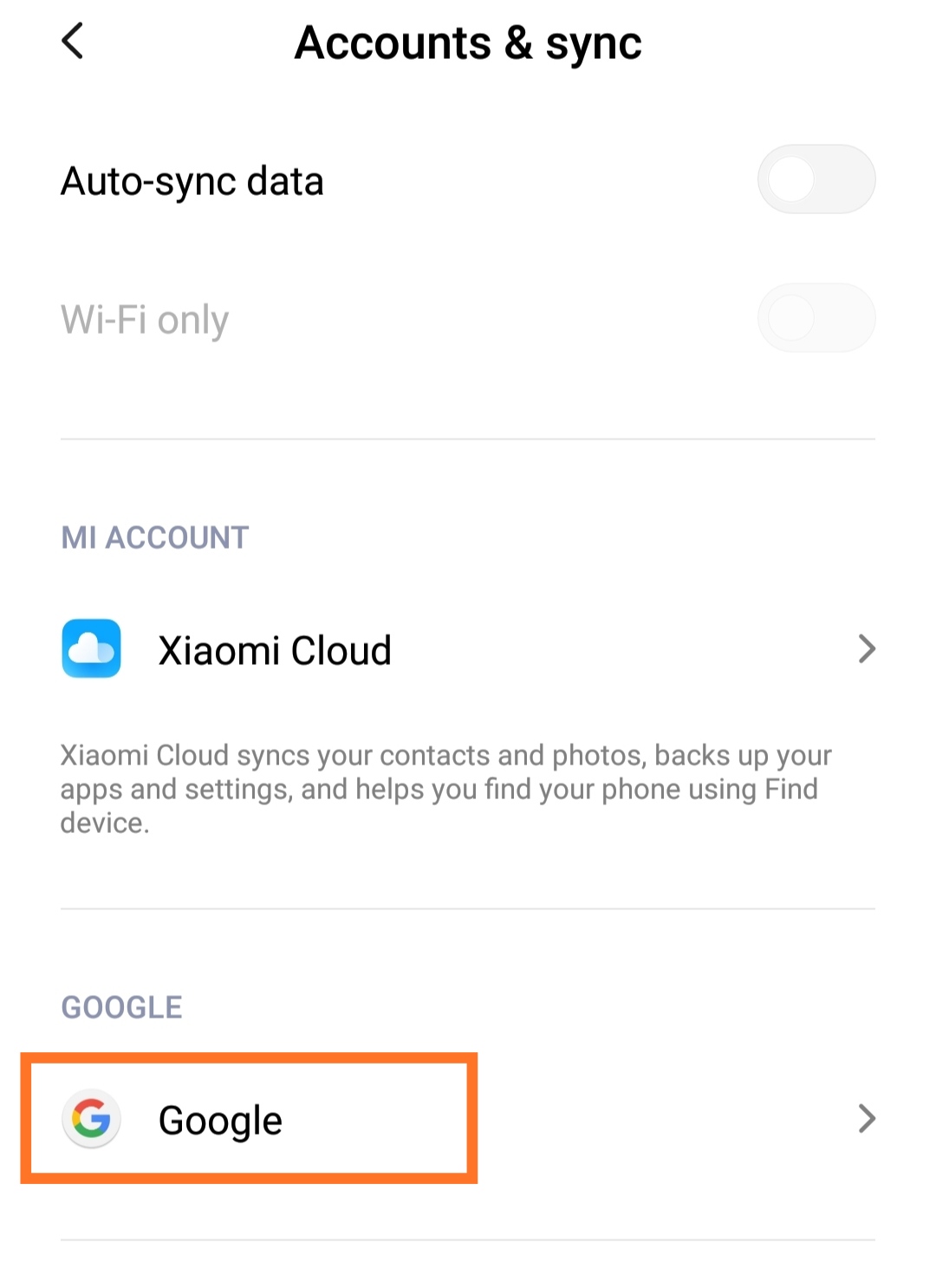This is a screenshot of a device settings menu, specifically the 'Accounts and Sync' section. 

At the top left, there is an arrow icon pointing to the left, indicating a back navigation option. Centered at the top, the title 'Accounts and Sync' is prominently displayed in bold black letters.

Directly below this title, aligned to the left, the option 'Auto-sync data' is listed. On the right side of this line, there is a toggle switch that is currently turned off. Under the 'Auto-sync data' option, in lighter colored text, 'Wi-Fi only' is mentioned.

Beneath these options, there is a larger box labeled 'My Account MI.' To the left of this label, there is a blue square icon. Below 'My Account MI,' it mentions additional functionalities: syncing contacts and photos, backing up apps and settings, and assisting in locating your phone number and devices.